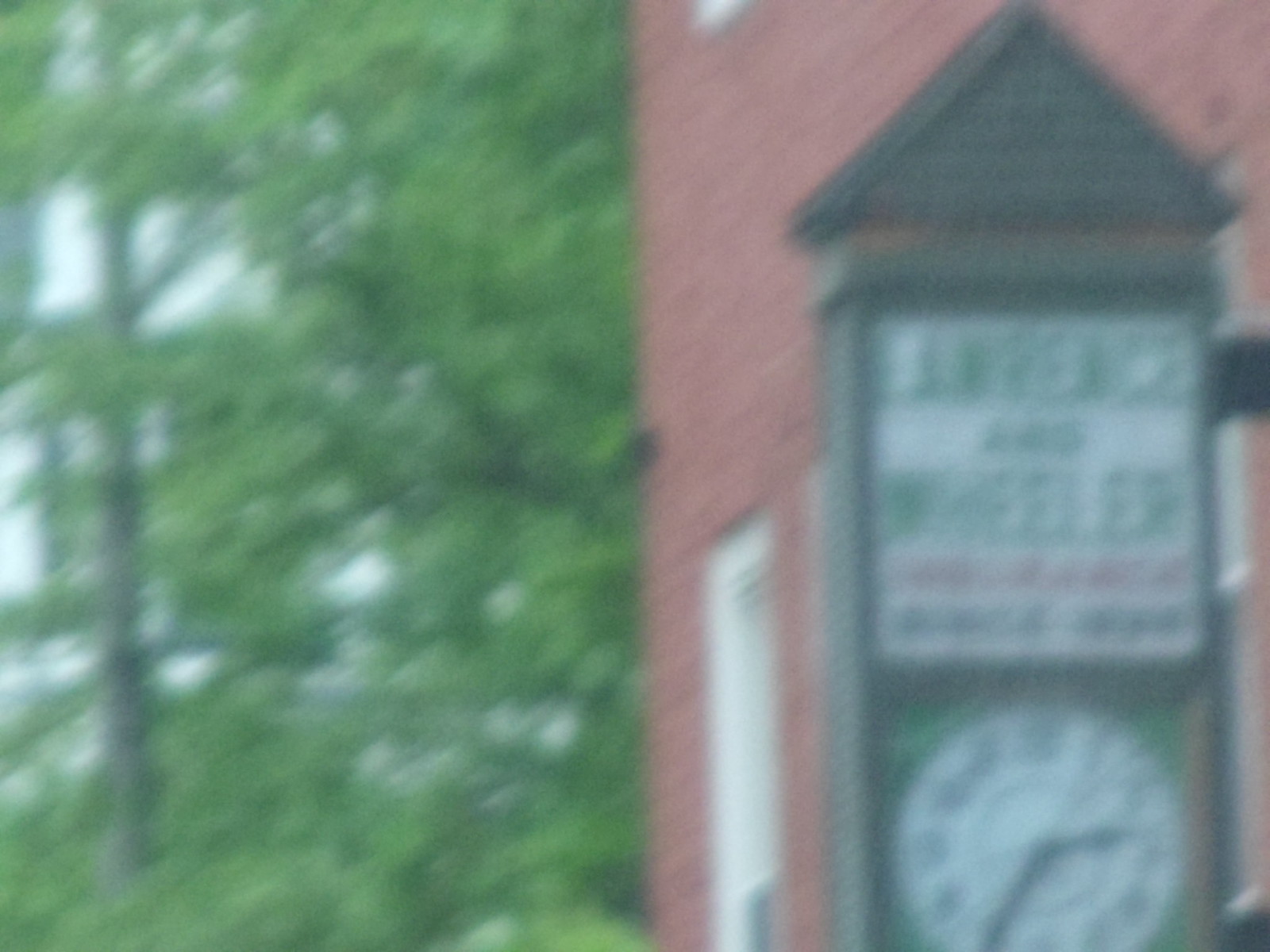The photo features a somewhat blurry image of a clock tower, which is part of a larger advertising billboard. Situated on the left side of the image are tall trees with a mix of branches and leaves, set against a gray sky. To the right, there's a red brick building adorned with white window trim. From the visible portion, the building appears to be at least two stories high, with part of an upper window and a fully visible lower window in the frame.

The focal point of the image, the clock tower, has a small roof-like structure on top. The advertisement above the clock is primarily in green text on a white background, although the exact wording is indiscernible due to the blur. Below the green text, there's some red text, which is also unreadable, followed by additional black text, all set against the same white background. Below this advertisement banner is the clock itself, which shows the time as approximately 2:35. This clock features black hands and black markings against a white face.